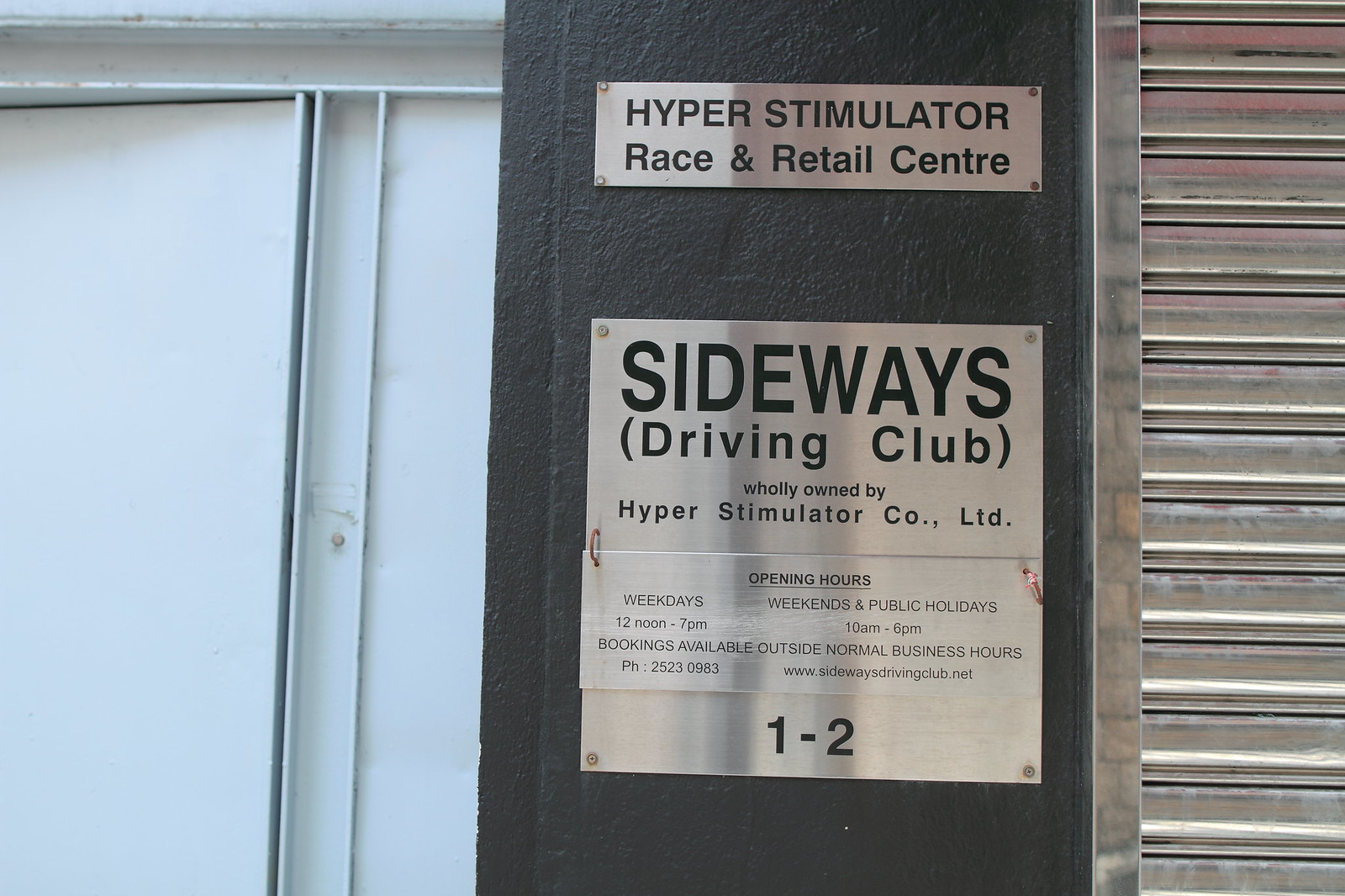This image captures a section of a black wall adorned with two stainless steel placards positioned centrally. The top, a horizontal rectangular sign, reads "Hyper Stimulator Race and Retail Center" in black lettering. Below it, a larger vertical sign states "Sideways Driving Club, wholly owned by Hyper Stimulator Co., Ltd." This lower sign also details the opening hours: weekdays from 12 noon to 7 pm, and weekends and public holidays from 10 am to 6 pm, noting that bookings are available outside normal business hours. Additionally, it provides contact information: a phone number (25230983) and a URL (www.sidewaysdrivingclub.net). At the bottom, the unit number "1-2" is prominently displayed. To the right of these signs, there is a distinctive pink and gray striped shutter, reminiscent of a house shutter or some type of metal rolling gate. To the left, the wall transitions into a white aluminum or light gray section, featuring vertical and horizontal I-beams, with a door seemingly opening on the far left.